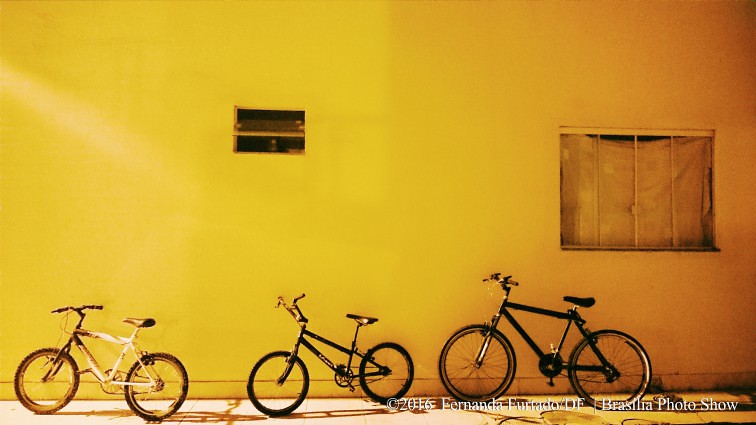This vibrant photograph, taken in 2016 and credited to Fernanda Furtado ©, captures an outdoor scene illuminated by sunlight filtering in from the left. The focus of the image is a striking, large yellow wall with three bicycles leaning against it, each contributing to a rich narrative of everyday life. The bikes, ranging from a small white child's bike with a narrow seat, a mid-sized girl's bike with taller handlebars, to an adult male's bike with a black seat and flat handlebars, all face left. Positioned close to the wall's right side is a larger window with three vertical white bars and a sheet hanging behind it, hinting at a homey interior. Above this, a rectangular cutout, functioning as a vent or smaller window, can be seen slightly offset to the left. This detail-rich setting is further enhanced by the brightly colored wall and the artist's signature at the bottom right, affirming its place in the Brasilia Photo Show.